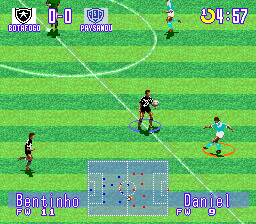The image is a screenshot from a pixelated video game depicting a soccer match on a field with alternating dark green and light green horizontal stripes and white markings typical of a soccer field. Five players are visible: three in dark uniforms (possibly black) and two in light bluish-green uniforms. A player in the center is marked with a blue circle underneath, indicating team affiliation, while a nearby player has a red circle beneath them. The upper right-hand corner shows a time of 4:57, and the upper left-hand corner displays a score of 0 to 0. At the bottom, the names "Bentino" and "Daniel" are shown with an overhead view of the field featuring blue and red dots representing the players between the names. Diagonal and partial circle white lines are also visible on the field, enhancing the scene's detail.